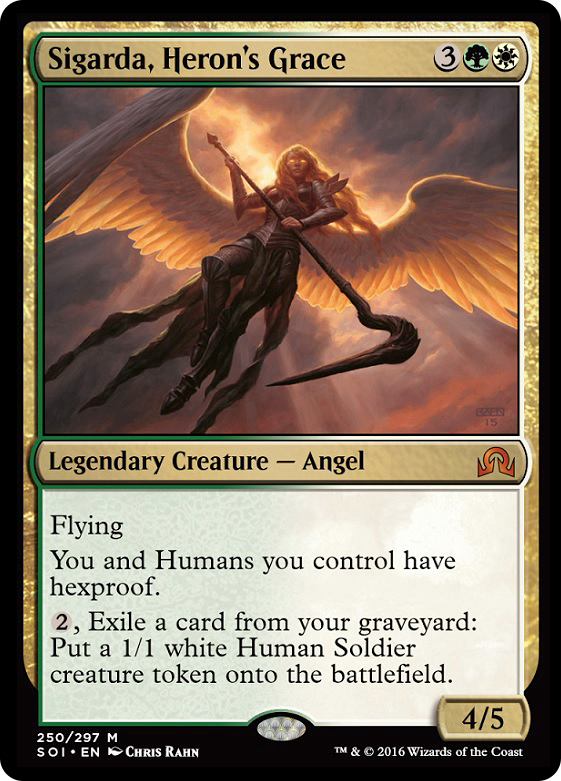The image depicts a card that appears to be from a collectible game, and it might be either a physical card or a digital representation on a screen. The card's title, situated at the top, reads "Sigarda, Heron's Grace." The artwork features an angelic creature with a human-like upper body and possibly a horse-like lower body, holding a long, slender staff that widens slightly before curving into a shape that resembles an upside-down bird's head. 

Beneath the illustration, the text categorizes the character as a "Legendary Creature - Angel." The abilities listed include "Flying" and "Hexproof" for both the user and the humans they control. Another ability requires the expenditure of two resources and the exiling of a card from the graveyard to generate a 1/1 white Human Soldier creature token on the battlefield. At the bottom of the card, it displays its power and toughness values as "4/5."